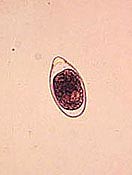The image is a detailed drawing of a single, isolated cell, resembling what one might see under a microscope. The cell, depicted in an oval shape with a small protrusion on top, features a prominent, dark red circular structure inside, likely representing the cell’s organ. This red structure is composed of tiny red dots with small black borders. The cell's outer membrane is tan-colored. The background of the image is a uniform peach color, adorned with various small, see-through bubbles. No other objects, text, or figures are present in the rectangular image, which has a longer width compared to its height.